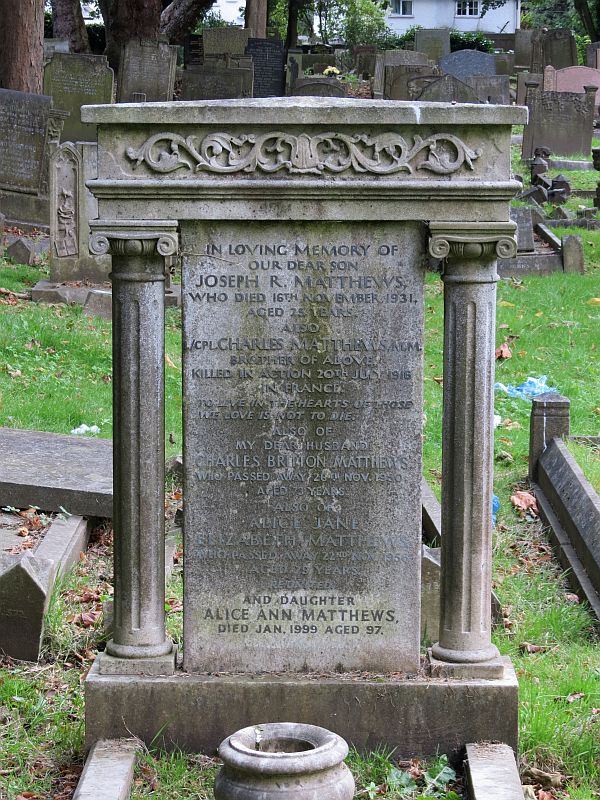In this realistic outdoor photograph, taken during a sunny day in a cemetery, the focus is on a prominent gravestone situated a few feet from the photographer. The scene includes green grass and a backdrop of trees and a white house. Among the 10 to 20 gravestones, mostly made of gray cement or stone, one stands out with its intricate design featuring two supporting columns and a carved top. This gravestone, though weathered and slightly discolored, is inscribed with the dedication, "In loving memory of our dear son Joseph R. Matthews who died in November 1931 aged 25 years." Beneath this, there are mentions of Corporal Charles Matthews, who was killed in action on July 20, 1916, in France, and of Alice Ann Matthews, who died in January 1999 at the age of 97. The details are enhanced by dark, chiseled lettering, although some parts have become difficult to read over time due to dirt and moss.